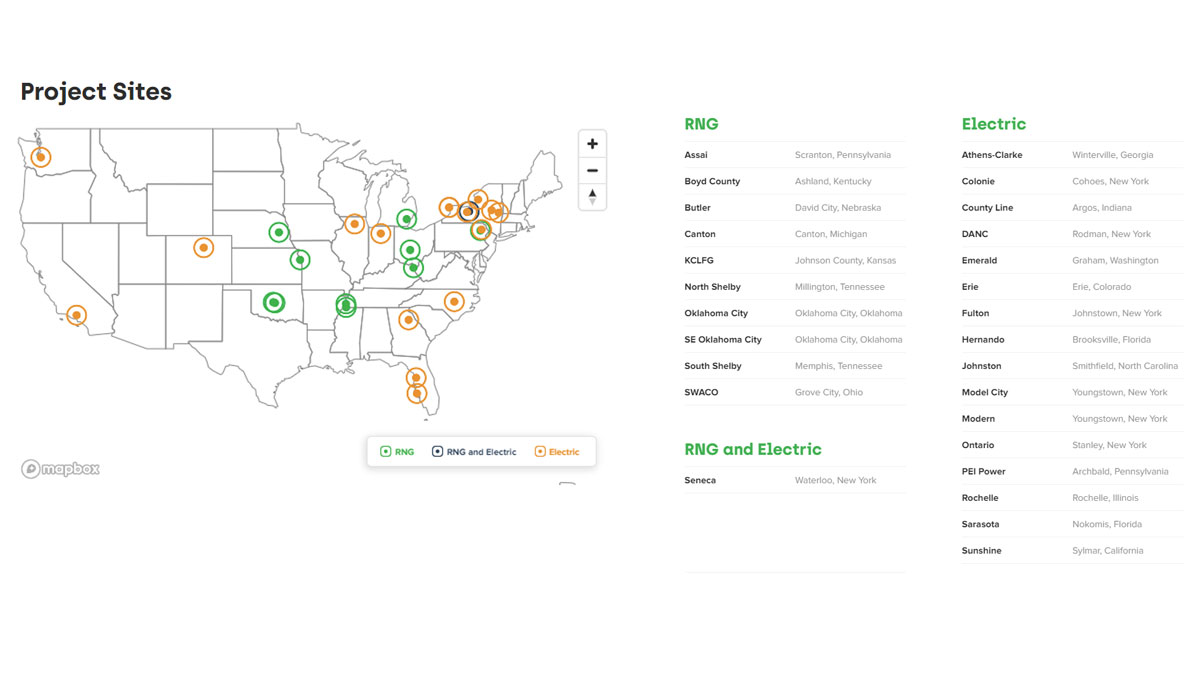The image showcases a detailed spreadsheet and map for a utility and infrastructure company specializing in natural gas and electricity management. Set against a white background, the left side prominently features a map of the United States marked with various orange and green dots. The orange dots represent electric sites that the company has managed or constructed, while the green dots denote RNG (Renewable Natural Gas) sites. There are approximately 30 dots scattered across the country, with a majority being orange and a few green.

On the right-hand side, the screen displays two vertical columns listing the active projects managed by the company. The first column is dedicated to RNG and combined RNG and electric sites. It features green headers labeled "RNG" and "RNG and Electric." Under the "RNG" header, there are about ten rows, each detailing different project sites in bold with their locations in light gray text. For example, an RNG site is listed in David City, Nebraska. The "RNG and Electric" section contains a single entry: the Seneca site located in Waterloo, New York.

The second column is titled "Electric" in green text, mirroring the format of the previous column. It lists approximately 15 electric project sites. Each entry includes the site's name in bold black text and its location in gray text, providing a clear and organized overview of the company's electric project locations.

At the top left, just above the map, the title "Project Sites" is prominently displayed in large black text, summarizing the image's focus.